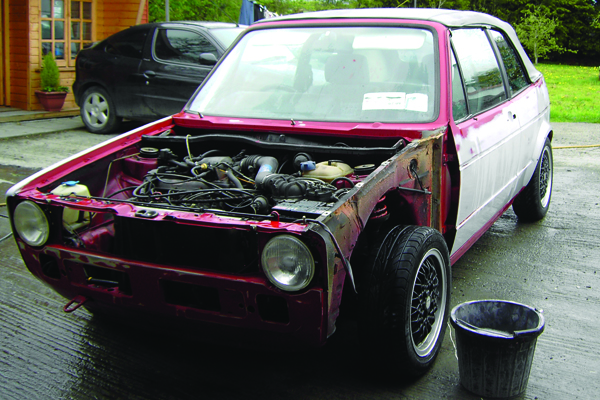This horizontally oriented outdoor photograph features an old convertible car, primarily painted white with some red metal areas exposed, indicating a possible past paint job. The car's hood and front bumper are removed, offering a clear view of its engine compartment, filled with a tangled mess of wires. The small round headlights remain intact on either side of the front. All windows are still on the car, and the top appears to be covered with a fabric, possibly a tarpaulin. The car's small tires are visible on each side. Beside the front tire, a bucket sits on the concrete surface. To the left, a more well-maintained car is partially visible, parked next to a brown building.